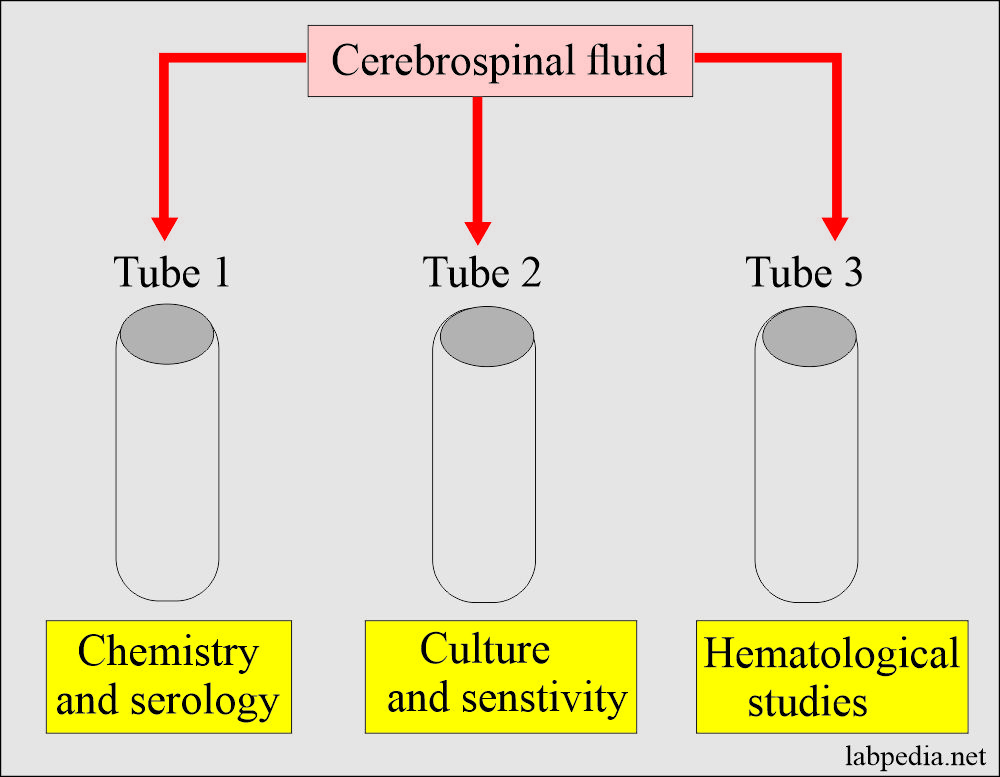The diagram, set in a landscape format, features the title "Cerebrospinal Fluid" prominently displayed in a light pink box at the top. Three red arrows descend from this box, pointing to three labeled sections: Tube 1, Tube 2, and Tube 3. Each label leads to a rough illustration of a test tube, characterized by a gray circle at the top and a cylindrical shape beneath it. Below each test tube, there are three yellow boxes, each containing distinct text: "Chemistry and Serology" under Tube 1, "Culture and Sensitivity" under Tube 2, and "Hematological Studies" under Tube 3. The background of the diagram is gray, and the bottom left corner features the website labpedia.net.